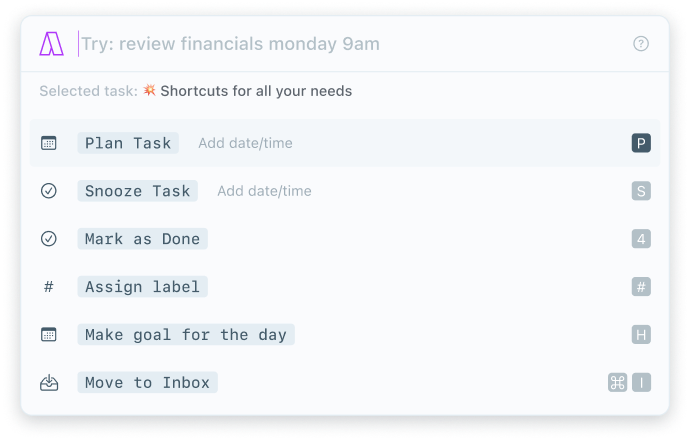**Caption:**

The image features a minimalist interface set against a very light gray backdrop. On the left side, an intricate letter "A" is illustrated, composed of multiple angles and lines. The "A" starts from the top, descends to the left, moves horizontally, angles upward to the right, then downward, moves horizontally again, ascends, and finally connects back to form the letter, with an additional diagonal line through its middle.

To the right of the "A," a thin vertical line splits the space, leading to text that reads "Grayish Try Review Financials Monday, 9 a.m."

On the far right side, there's a circle featuring a crest marked in gray. Below the "A," a thin horizontal line is followed by the text "Selected Task" in gray. Under this, a small yellow center with red sparks emanates, while the phrase "Shortcuts to All Your Needs" is displayed in black.

Running down the left side are six icons representing different tasks, each with corresponding descriptive text to the right. These are listed as follows:
1. Calendar
2. Plan Task
3. Add Date/Time

On the right side, from the top down, there is a sequence of shapes and letters:
1. Dark blue square with a "P"
2. Light gray square with a check mark labeled "Snack, Snooze Task"

This alternating pattern continues all the way down:
- "Marker's Drone"
- "Assign Label"
- "Make Goal for the Day"
- "Move to Inbox"

Further down on the right side, matching these tasks, are light gray squares sequentially marked with an "S," "4," "#," "H," "I," and another "H" with small circles on the tips. All lettering on the interface is white, maintaining a clean and monochromatic aesthetic.